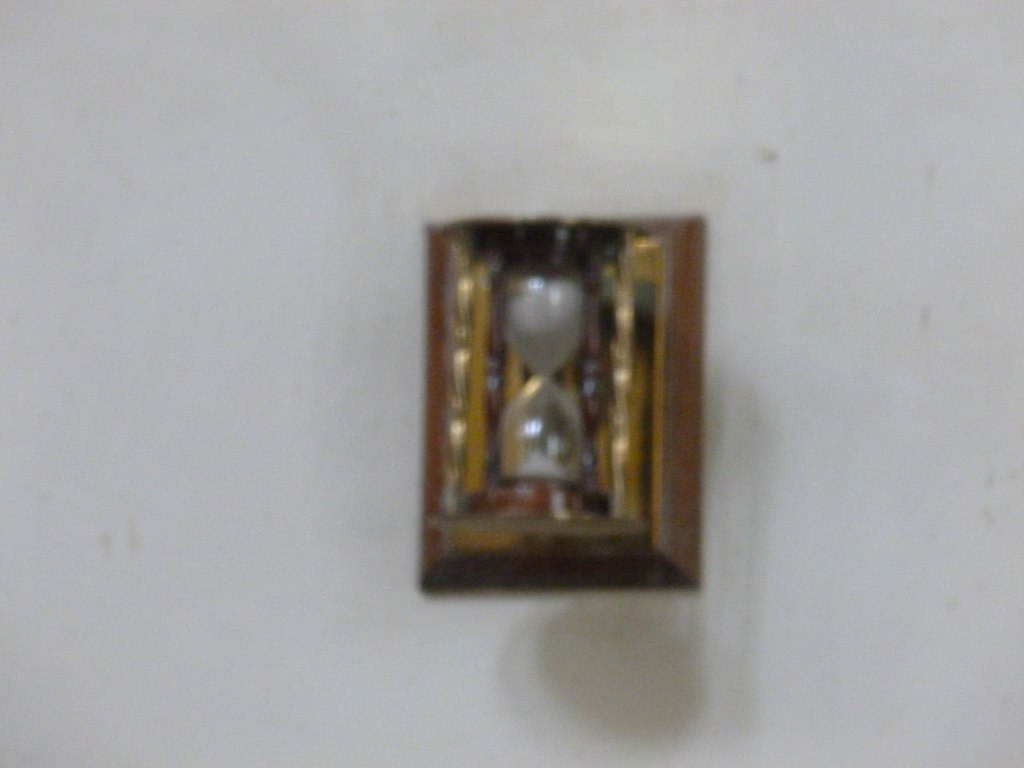This is a very out-of-focus photograph of what appears to be an old-fashioned hourglass enclosed in a rectangular, wooden-framed case with gold or brass accents. The hourglass features predominantly white sand, mostly accumulated at the top, with only a small amount having passed through to the bottom. The object seems to be presented as though it could be an artifact or museum piece, possibly a modern replica. The case holding the hourglass has a distinctive structure with a mix of metal and wood elements. The background of the image is a grayish-violet wall, and there is a noticeable shadow cast by the hourglass and its case onto the wall. The piece is relatively small and features a round, wooden base.